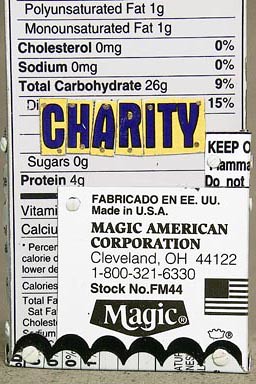The image is a color photograph featuring a detailed, multilayered label composition. The primary element is a nutritional label with a white background and black text. The label includes information on polyunsaturated fat, monounsaturated fat, cholesterol, sodium, total carbohydrates, sugars, and protein, each followed by their respective percentages. This label appears to be slightly cut off and occupies most of the photo, set against a medium grey background towards the lower edges.

Prominently overlaid in the middle is a small, torn yellow label with the word "CHARITY" handwritten in blue pen. The text is in a large, dark blue, bubble-style font, and appears slightly jagged at the bottom as if it had been cut or torn out.

Below this yellow label, towards the bottom right, is another white rectangular tag with black text that reads "Magic American Corporation, Cleveland, Ohio." Adjacent to this, on the right side, there is a black logo of an upside-down crown with the word "MAGIC" inscribed in white and a representation of the American flag without stars. Additionally, a series of curved black and white lines are drawn at the very bottom of the image, which appears to comprise multi-layered documents made from various pieces of paper.